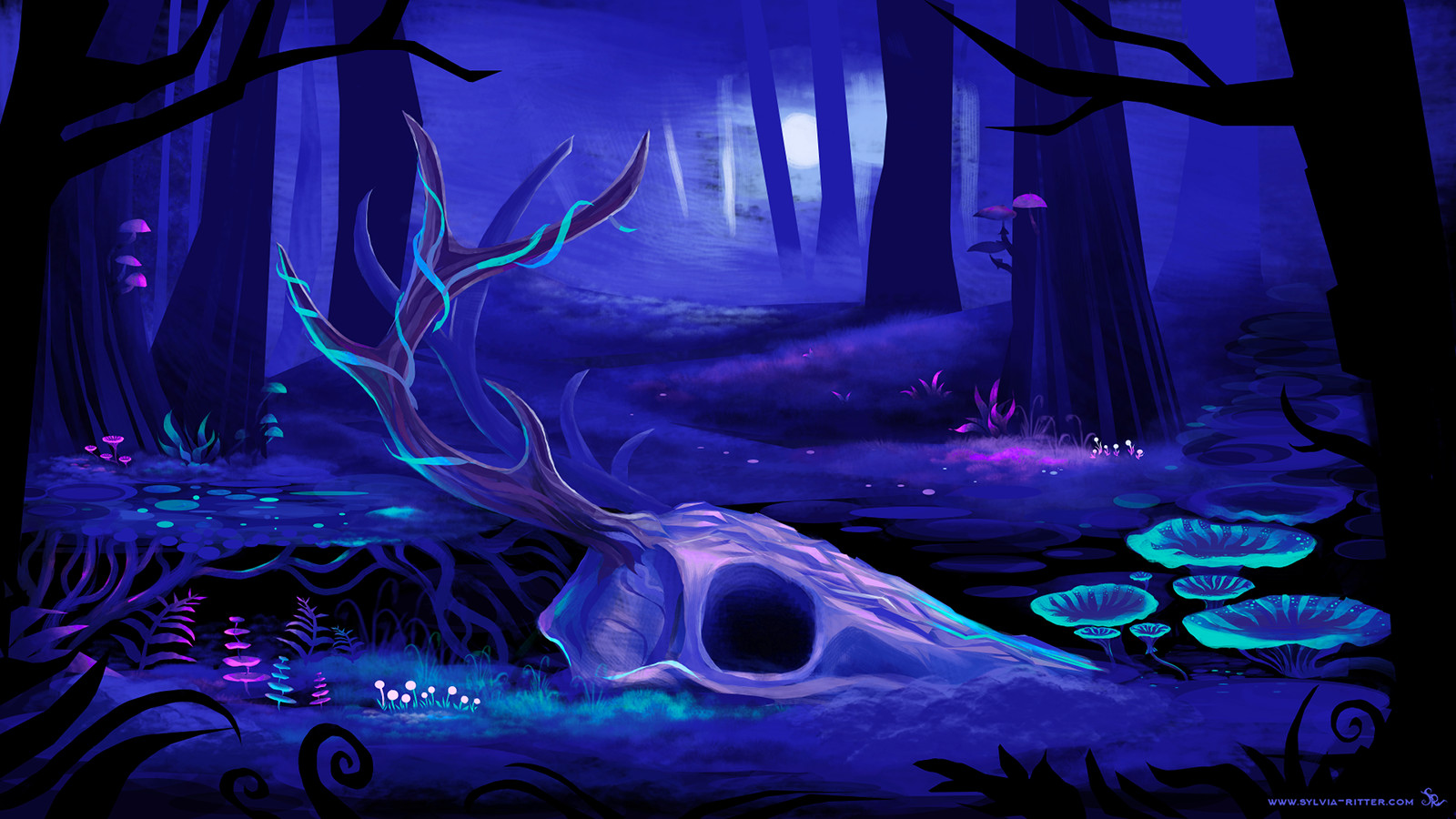The image portrays an animated scene set in a forest at night, characterized by a pervasive dark blue hue. Illuminated by a moonlight filtering through the trees in the distance, the scenery reveals various glowing flora. Prominent in the forest are glowing mushrooms in shades of green and pink, and equally luminous flowers and plants in pinks and yellows, scattered around the tree trunks. Notably, some of these glowing plants resemble ferns and even small Christmas trees.

Amidst this bioluminescent environment, a significant feature stands out: the partial skull of a large creature at the center of the image. This skull, likely belonging to a deer or bull, prominently displays large, intricate antlers extending upward and outward. The skull itself does not glow, but it is illuminated by the surrounding bioluminescent flora, giving it an eerie yet enchanting appearance.

The forest background includes several trees with trunks extending out of the frame, their black branches adding to the dark, mysterious ambiance. The ground, covered in dark grass and adorned with scattered flowers and plants, appears to have a blue tint reflecting the overall color scheme of the setting.